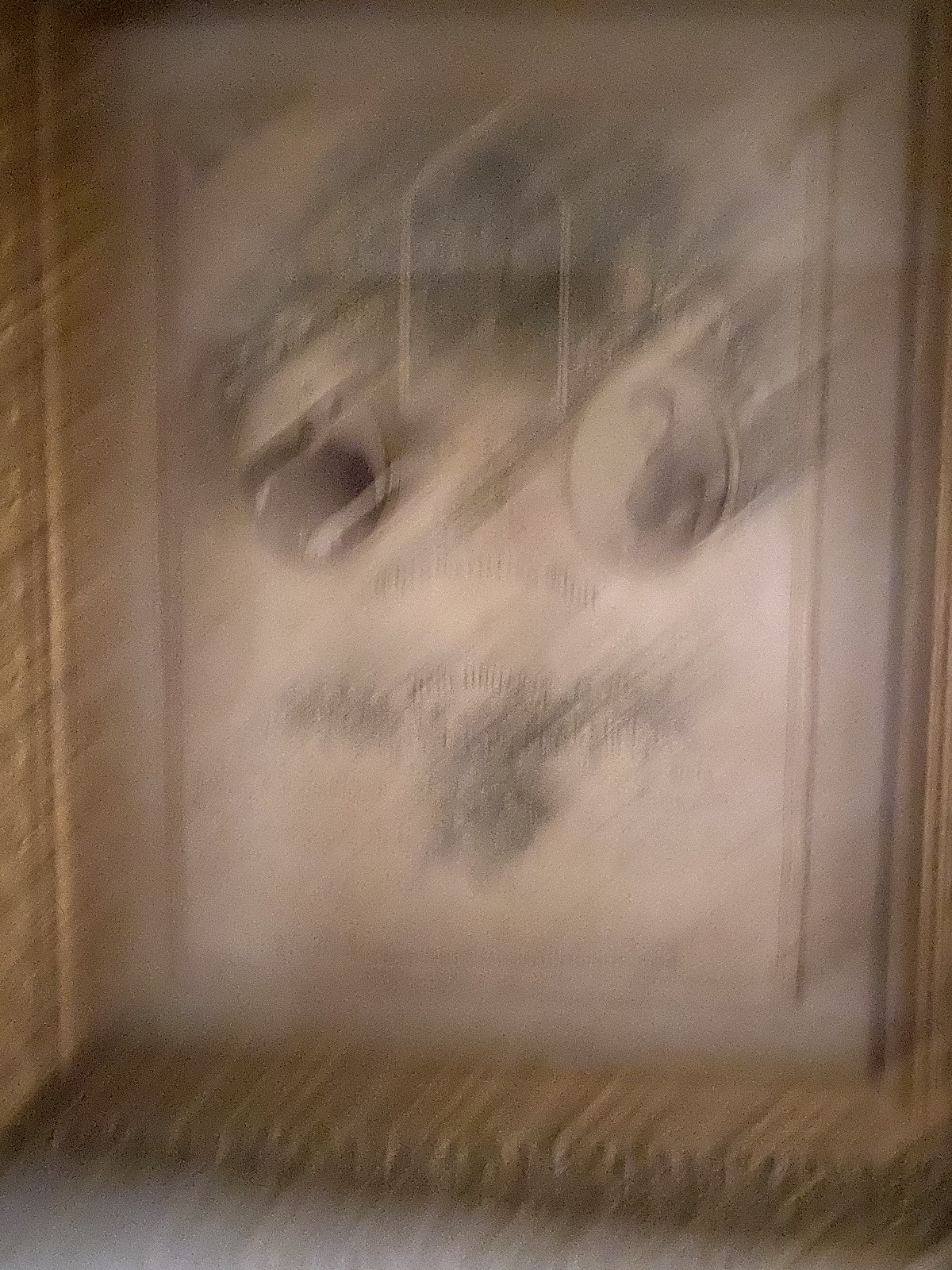This image features an extremely blurred and likely intentionally obscured, black-and-white framed picture comprising three distinct sections. At the center, there are two prominent oval-shaped portraits: on the left, an old-time image of a man staring directly into the camera, and on the right, a woman who is positioned with her body facing left but with her head turned towards the camera. Both portraits embody an antique aesthetic. Above and centrally-aligned between the two ovals is a chapel-like shape, which is difficult to discern, but may depict a building with trees. There's an arched inscription below these images in old English styling, further adding to the vintage look. The overall framing and content hint at a nostalgic, possibly historical significance, though the heavy blurring makes detailed interpretation challenging.